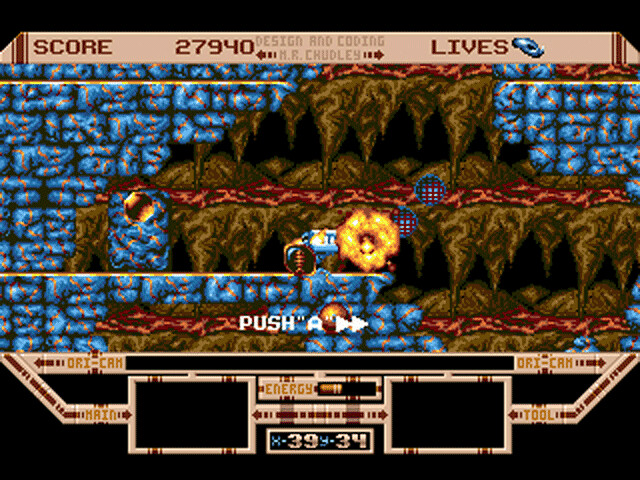This image depicts a screenshot from a video game, likely played on a console or PC rather than a cell phone. The game features a visually striking design with intricately carved blue cube blocks that dominate the left-hand side and stretch over the top towards the center. The upper right corner also showcases more of these blue cube blocks. The background is predominantly black, adding contrast to the vibrant in-game elements. Across the top of the screen, there's a tan banner with dark brown accents at either end, displaying the score of 27,940 and indicating one remaining life. 

At the bottom center of the screen, the text "PUSH A" is highlighted in white, flanked by two arrows pointing right. Just above this message, perched on a blue brick ledge, is a blue machine or robot. To its right, a large yellow fireball is in motion, suggesting a dynamic moment in gameplay. Underneath the main game window, additional information is displayed in a segment that includes numbers and terms like "ENERGY" with values "39" and "34". The detailed visuals and structured interface hint at a classic arcade or retro-style game, with precise design elements such as the note, “Design and Coding by M.R. Chuttles,” subtly included in the upper banner.